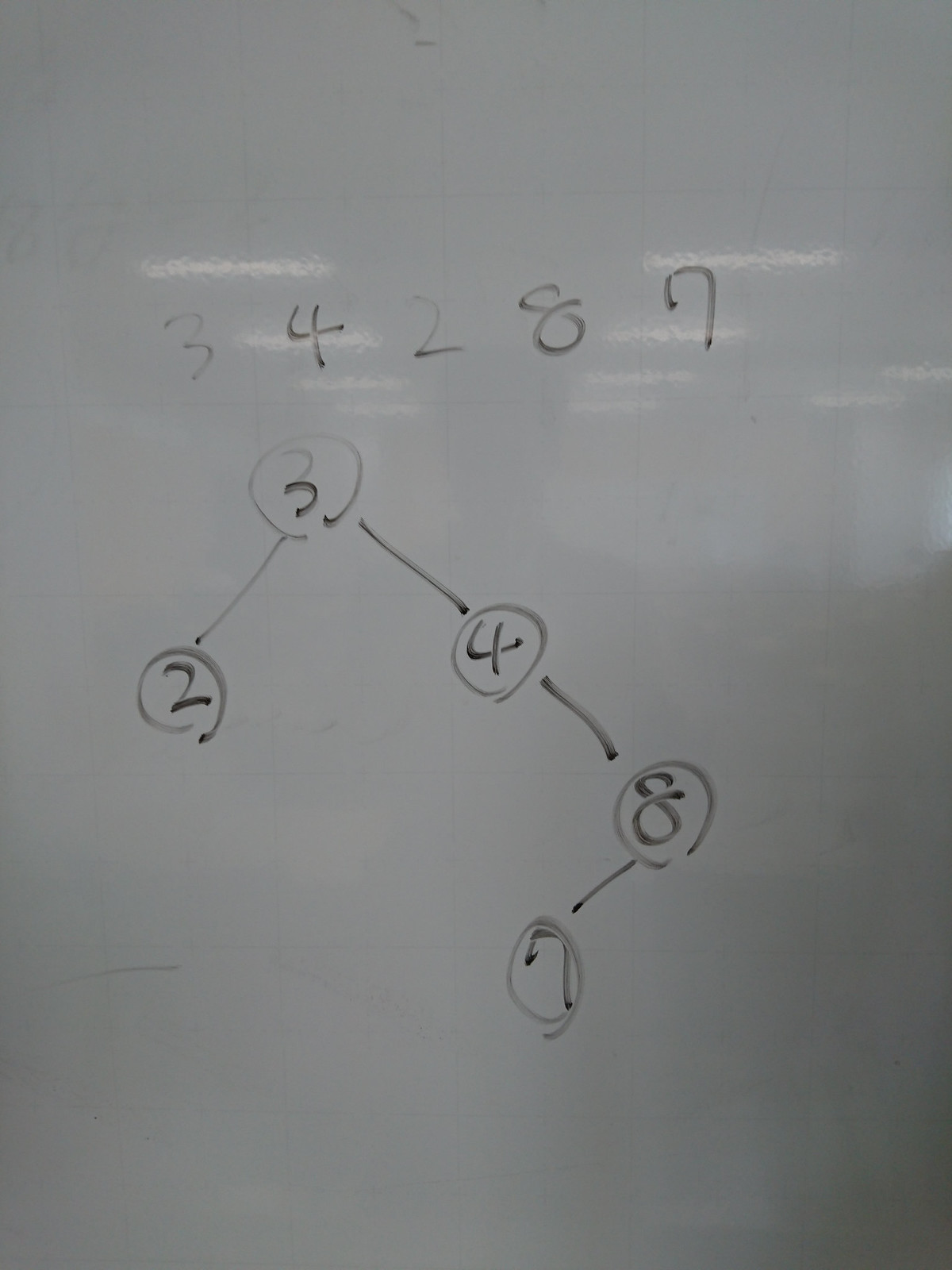In this image, a blurry and poorly lit photograph captures a dry erase whiteboard in a classroom setting. Due to the dim lighting, the whiteboard appears gray rather than its typical white color. The reflection of the classroom's fluorescent ceiling lights is visible on the board, revealing rectangular light fixtures and the silhouette of the person taking the photo, who is holding a phone. The content on the whiteboard includes faint black marker inscriptions. At the top, the sequence "3 4 2 8 7" is written. Below this, a simple graph is drawn, consisting of circles connected by lines. The graph features a circle labeled "3" at the top, from which lines extend downward. One line leads to a circle labeled "2" positioned to the lower left, and another line leads to a circle labeled "4" towards the lower right. From the "4" circle, a line descends to a circle labeled "8," and further down, another line connects to a circle labeled "7."